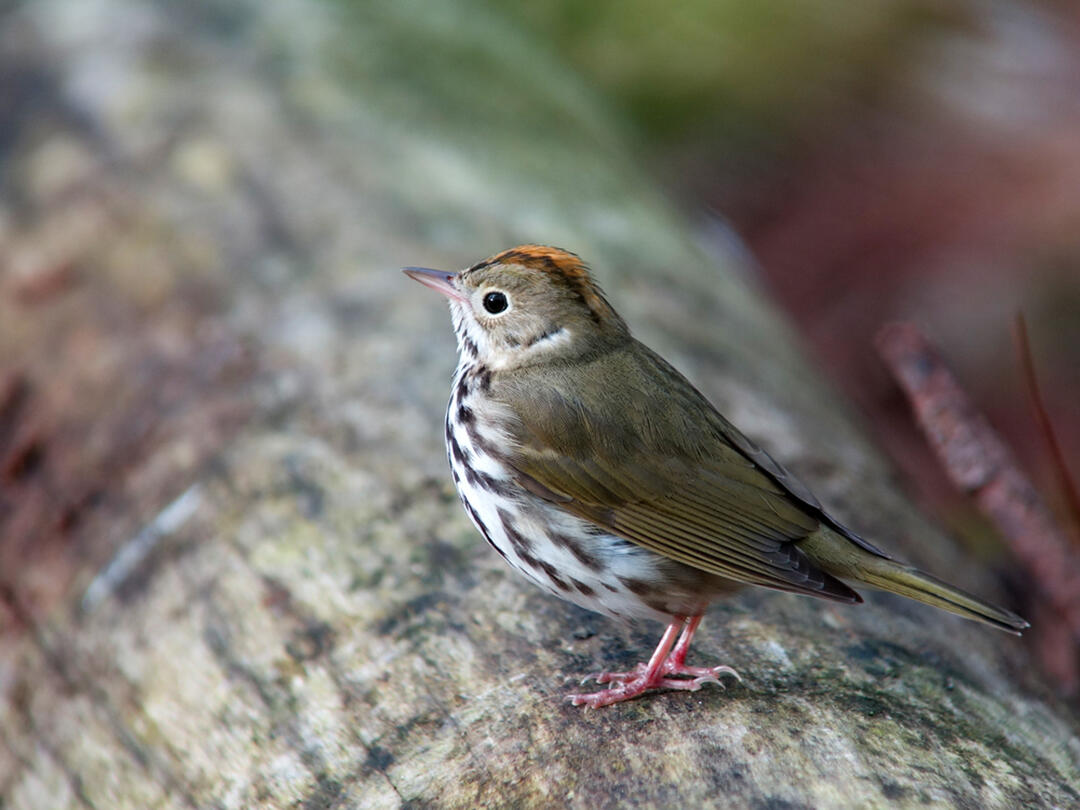The photograph captures a detailed and close-up side view of a small, plump bird perched on a large tree branch or piece of bark. The bird, which has a mix of light brown, orange, black, and dark green feathers, is looking up to the top left, clearly showing one of its black eyes. Its head feathers display a richer blend of colors, including light brown and black, while its belly is adorned with white feathers speckled with black and brown spots. The bird’s beak is a striking combination of pink and black, and its pink claws grip the branch securely. The tree branch, varying in shades from light brown to dark brown and black, is sharply in focus, contrasting with the blurry background, which emphasizes the bird as the central subject in this brightly lit and clear image.